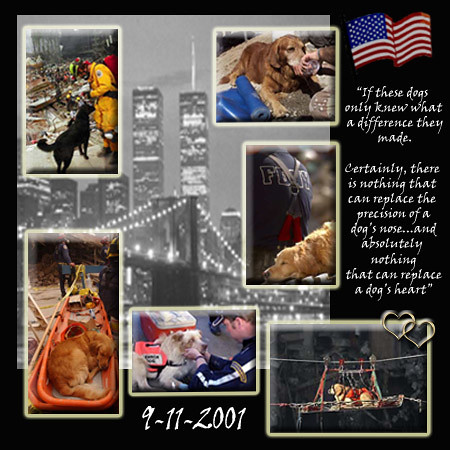This image is a detailed collage set against a gray, stenciled view of pre-9/11 New York City, prominently including the Twin Towers. At the bottom of the collage, the date "9-11-2001" is clearly displayed in white text. The collage features six pictures, each outlined in a vivid, LED-like white frame. 

Within these frames, images of dogs engaged in various acts of heroism are depicted. On the left, a vertical image shows a black dog resting beside a firefighter. Below this, another dog is curled up with some supplies, and next to it, a terrier-like dog has supplies strapped to its back while working alongside a rescue worker. In the middle, a large dog resembling a St. Bernard is being transported on a stretcher over what looks like a canyon. Above, a spaniel-type dog rests its head against a stone, possibly mourning its owner, and another spaniel is featured with supplies.

On the right side of the collage is a vertical image of an American flag. Beneath it, a heartfelt quote in scripted style reads: "If these dogs only knew what a difference they made. Certainly, there is nothing that can replace the precision of a dog's nose, and absolutely nothing that can replace a dog's heart." Interlinked metal hearts, resembling rings, are displayed beneath the text.

The overall composition acts as a tribute to the rescue dogs who played vital roles during the aftermath of the September 11 attacks, highlighting their irreplaceable contributions and the profound impact of their efforts.